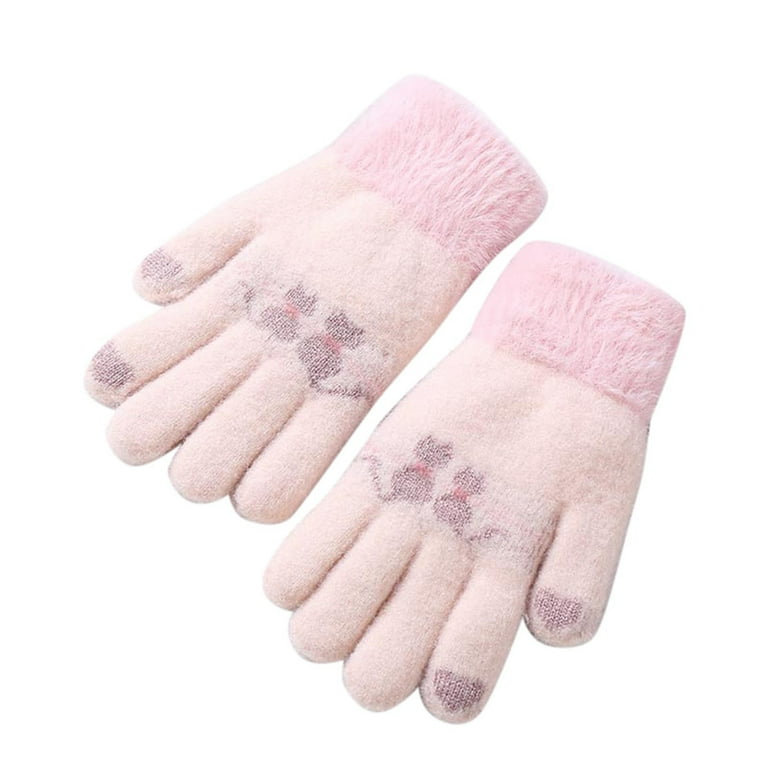This photograph showcases a pair of small, child-sized, pink mittens set against a white background. The mittens are soft and fuzzy with a simplistic design featuring playful elements. Each mitten is adorned with a silhouette of two black or gray cats with red collars, positioned by the fingers and extending towards the middle of the palm. The cats' tails are whimsically drawn, curving upwards. 

The fingertips of the thumbs and index fingers have special dark areas versus the rest of the regular pink, possibly designed for touch-sensitive device compatibility. The mittens also have vibrant, longer-fibered cuffs that are a slightly darker shade of pink, encircling the wrist area. The gloves are oriented with the fingers pointing down to the left, and the thumbs are on the outside, giving a clear view of the detailed patterns and textures. This combination of features suggests the mittens are not only cute but functional, aimed at young children who enjoy playful yet practical accessories.